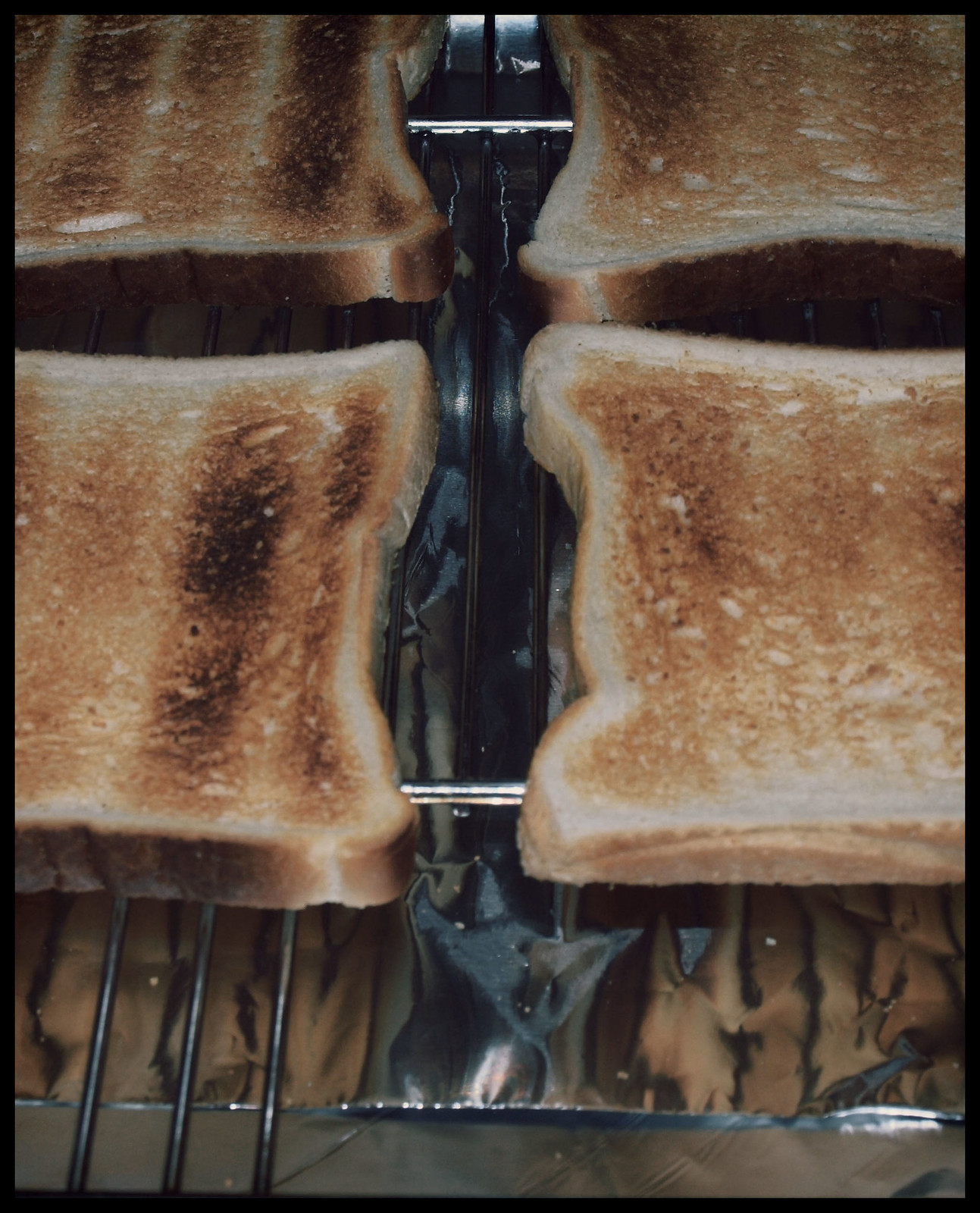This is an up-close photograph taken from above, showcasing four pieces of white bread that have been toasted to varying degrees, with some slices near burnt. The toast pieces are positioned in a cross formation with two slices on the top and two on the bottom. The image is partially cut off on both sides, so the left and right slices are only partially visible. The toast is resting on a metal grill rack inside what appears to be an oven, with a sheet of wrinkled aluminum foil beneath it. The foil reflects the metal bars and the toast. Grill marks indicate that the bread was likely flipped during toasting. The background is entirely composed of the metallic grill and aluminum foil, emphasizing the close-up, almost macro nature of the photograph.